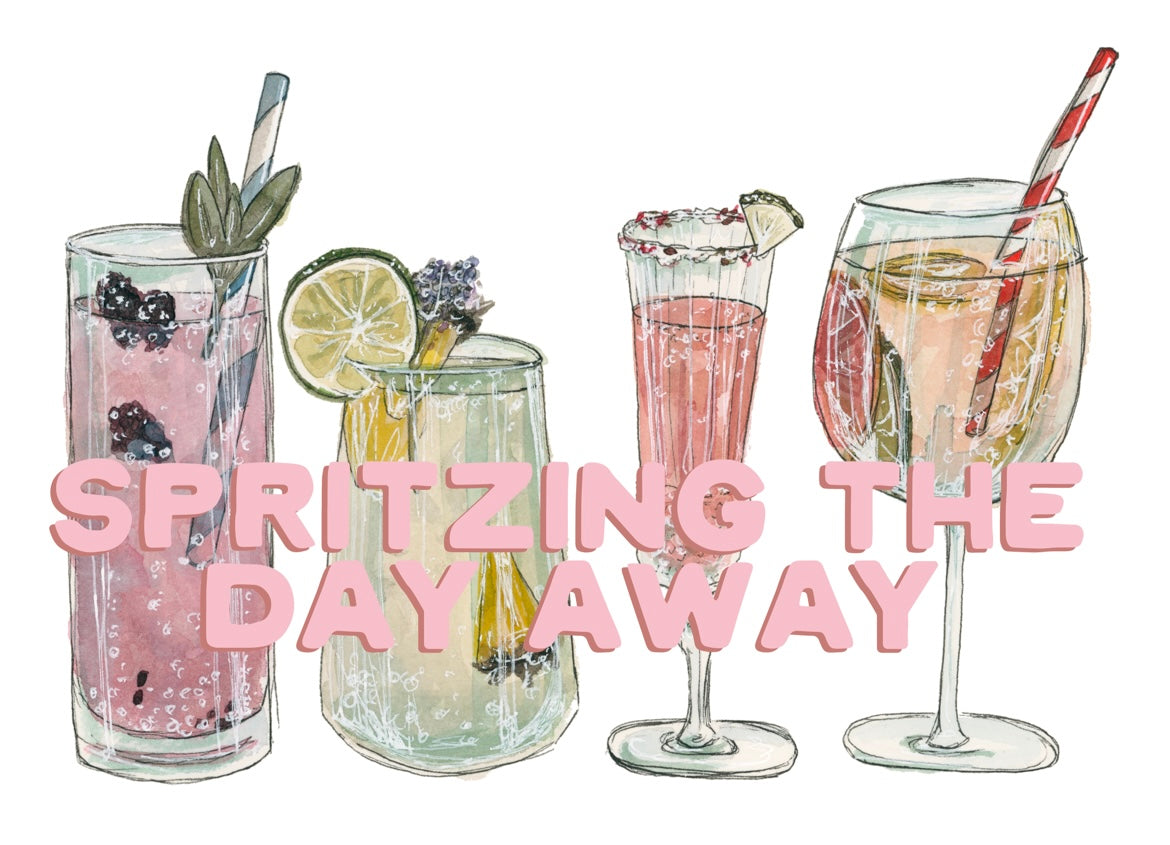The image features a colorful array of four illustrated spritzer drinks, each distinct in appearance but unified by an overarching theme. Bold, bright pink typeset across the front of the image reads "Spritzing the Day Away," suggesting a lively, refreshing atmosphere. From left to right, the first drink is a tall glass filled with a pink carbonated liquid, adorned with green leaves and berries, and accessorized with a blue and white striped straw. Next to it, a shorter, clear glass offers a yellowish-green drink with a lime slice on its rim and other floating elements, possibly berries. The third drink, resembling a champagne flute or a sundae glass, contains a pink liquid and has a rim encrusted with what appears to be sugar or salt, complemented by a lime slice. The final drink is a wine glass filled with a faint pink liquid and infused with multicolored fruits. This drink is finished with a whimsical red and white striped straw resembling a barber pole. The entire composition suggests a vibrant, playful take on these spritzer beverages.